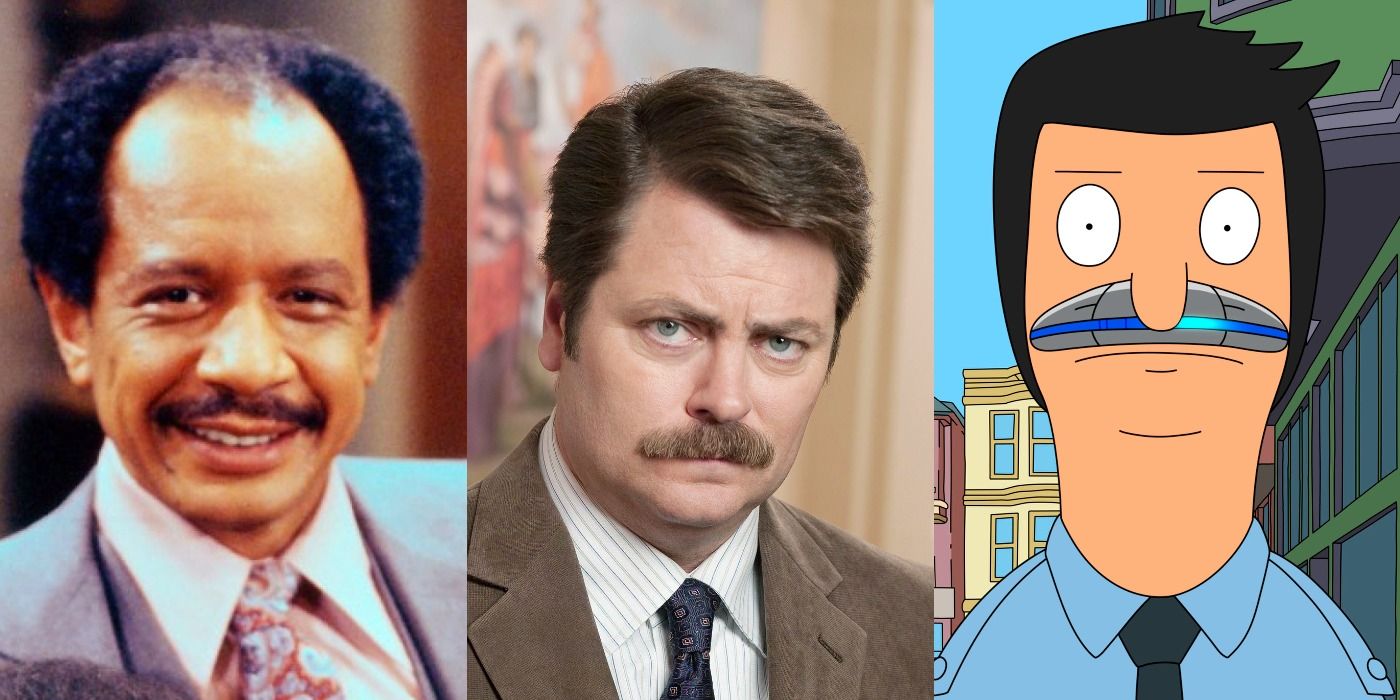This composite photograph features three distinct images of well-known TV characters. To the left, there is a photograph of Sherman Helmsley portraying George Jefferson from the classic 1970s TV show. He is an African American man with balding, poofy dark hair and a mustache, dressed in a gray suit with a white shirt and a floral tie, smiling brightly at the camera. In the center, Nick Offerman is seen as Ron Swanson from Parks and Recreation. He sports thick, dark hair parted to the side, a thick mustache, and a serious expression. He is dressed in a brown suit jacket over a white striped shirt with a blue tie, staring directly at the viewer. On the right, an animated depiction in the style of a cartoon character closely resembles Bob Belcher from Bob's Burgers. This cartoon figure, distinguished by his blue shirt, black tie, and an electronic device with a blue LED light strip in place of his usual mustache, has black hair and wide, oval eyes with small pupils. This array of images highlights three iconic characters from television, each rendered in a unique style and expression.